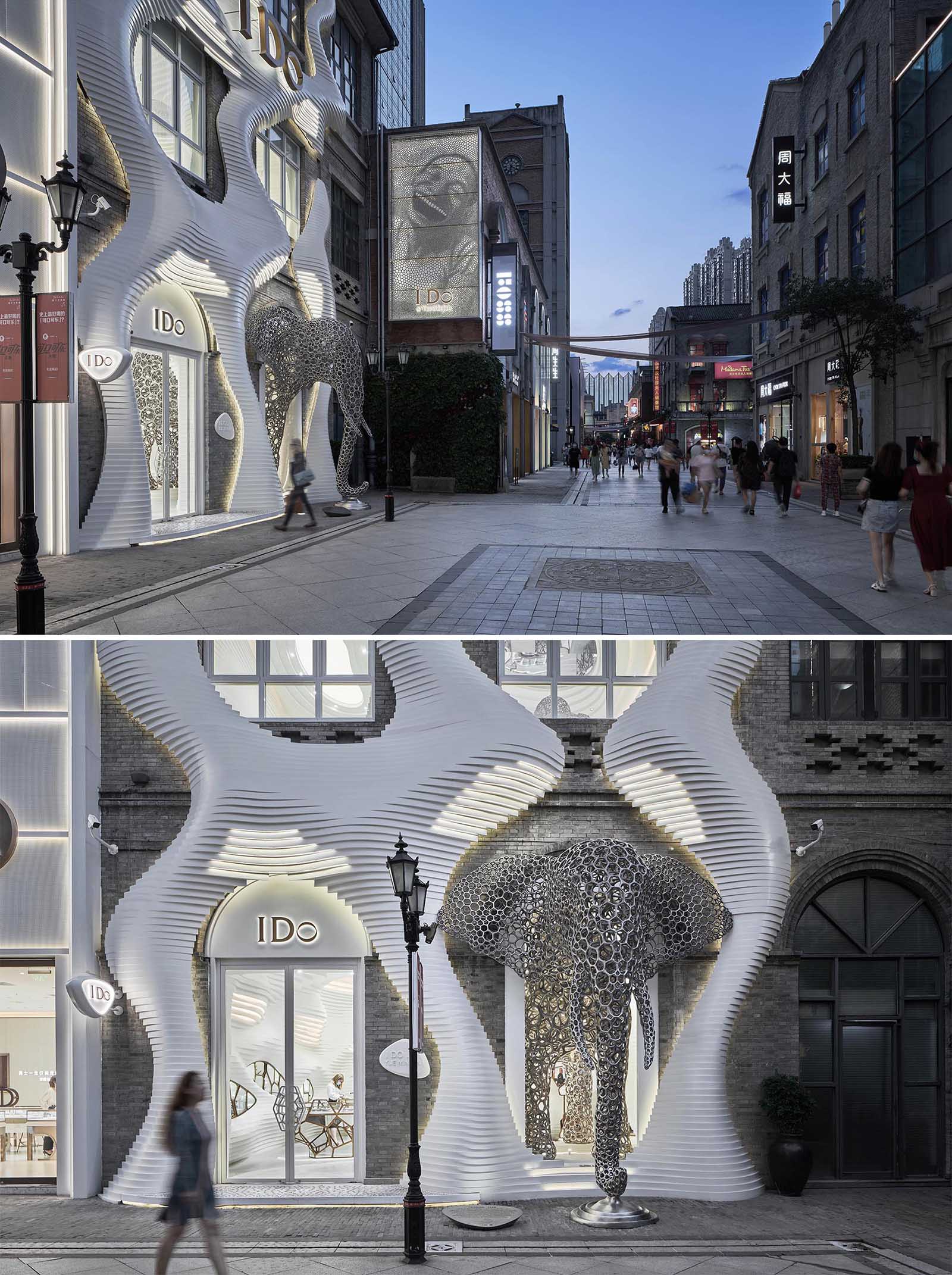This image is a composite split into two parts, depicting an urban street scene in what appears to be an Asian shopping district. The upper section provides a broad view of a bustling street lined with various storefronts adorned with Asian lettering in white on black backgrounds, suggesting a lively commercial area. Prominently featured is a unique building with an arched entrance labeled "I Do." Surrounding the entrance is a fascinating, wavy white modern art structure with noticeable hatches. The lower portion offers a closer, more detailed look at this intriguing building. Beside the entrance, there's an intricate metallic sculpture resembling the front of an elephant, crafted from silver chains, complete with tusks and a trunk that extends to the ground. The scene is animated with various pedestrians, including a blurred figure walking in front of the I Do store, emphasizing the everyday life and vibrant activity of the location.